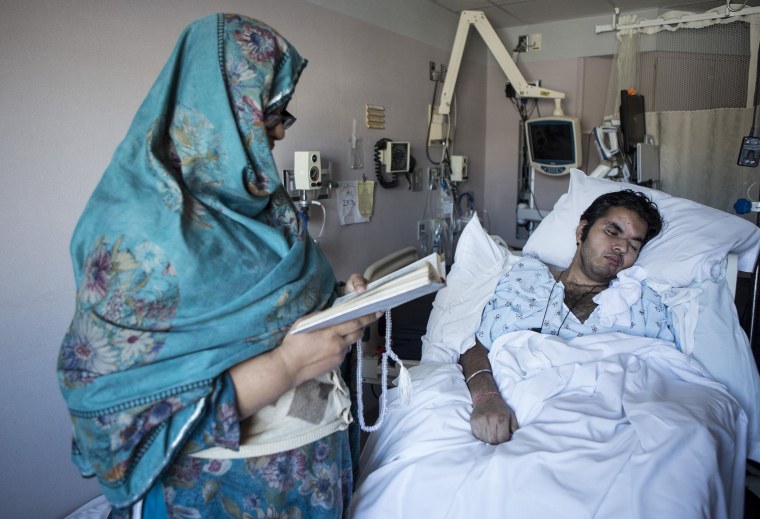In this detailed photograph, a man in his late 20s or early 30s is depicted unconscious in a hospital room, suggesting he is gravely ill or severely injured. He is dressed in standard hospital attire and lies under a white blanket with his head resting on a white pillow. His right arm is visible, placed atop the blanket, hinting at possible injuries to his face, arm, or hand. Surrounding the bed are various pieces of hospital equipment, including monitors and other medical devices for checking vital signs like blood pressure and heart rate, all typical of a hospital setting.

Standing to the left of the man's bedside is a woman whose serene presence contrasts with the stark clinical environment. She is dressed in a turquoise dress and a matching floral hijab, and she wears glasses. Her hands hold a book from which she appears to be reading, possibly religious texts or last rites. The walls of the room are a neutral tan color complemented by white trim, adding a subtle warmth to the otherwise sterile atmosphere. The woman's attire adds touches of blue, green, and a hint of orange, standing out against the predominantly white and off-gray tones of the hospital room.